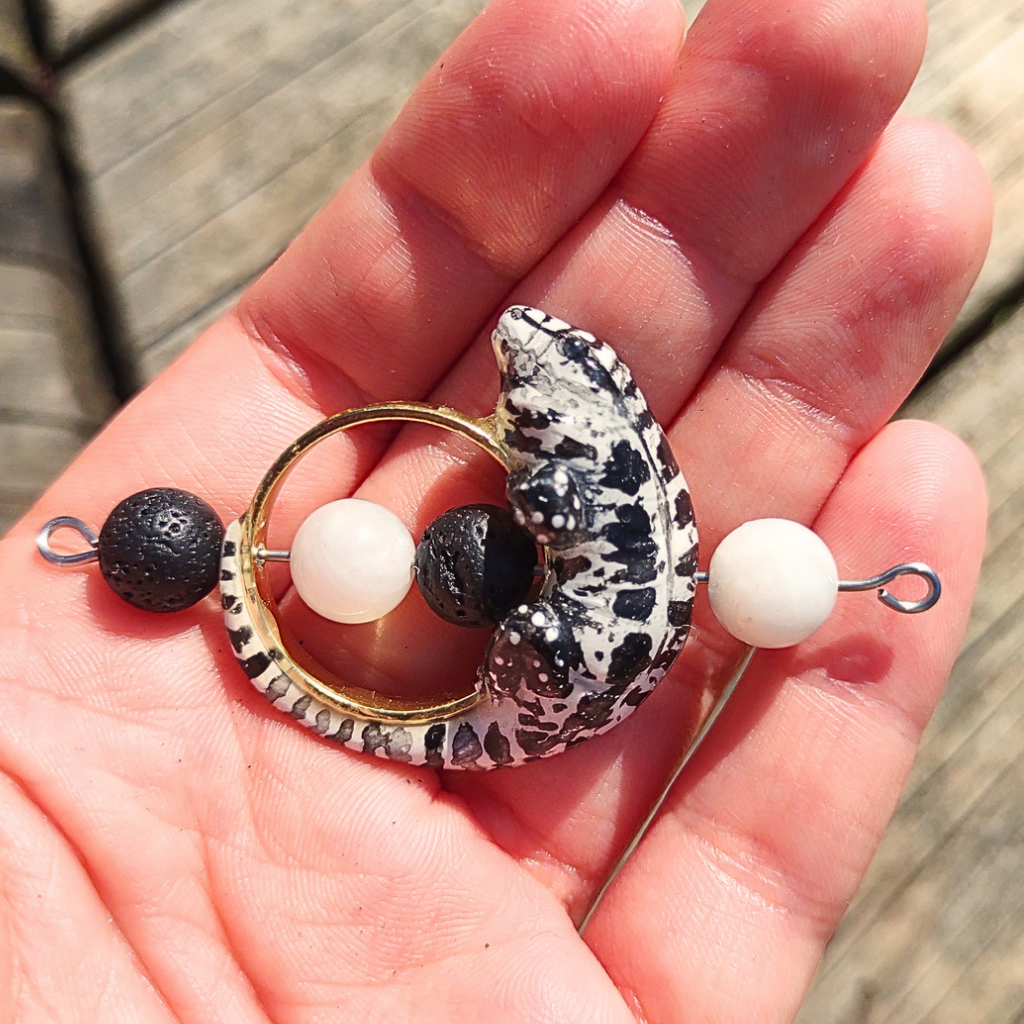This image showcases a detailed piece of jewelry, likely an earring or decorative pin, held in the palm of a person with a light complexion. The backdrop hints at wooden decking. The primary feature of this ornate piece is a central gold ring encircled by a black and white lizard, which wraps around the ring with its tail curling to the left. This lizard is intricately detailed with spots, squares, and stripes. A silver rod traverses through the middle of the gold ring, aligned with four textured balls—alternating in color between black and white. The order of the balls from top to bottom is black, white, black, and white, each appearing to have small indents. The arrangement and meticulous design suggest a high level of craftsmanship in this unique jewelry piece.